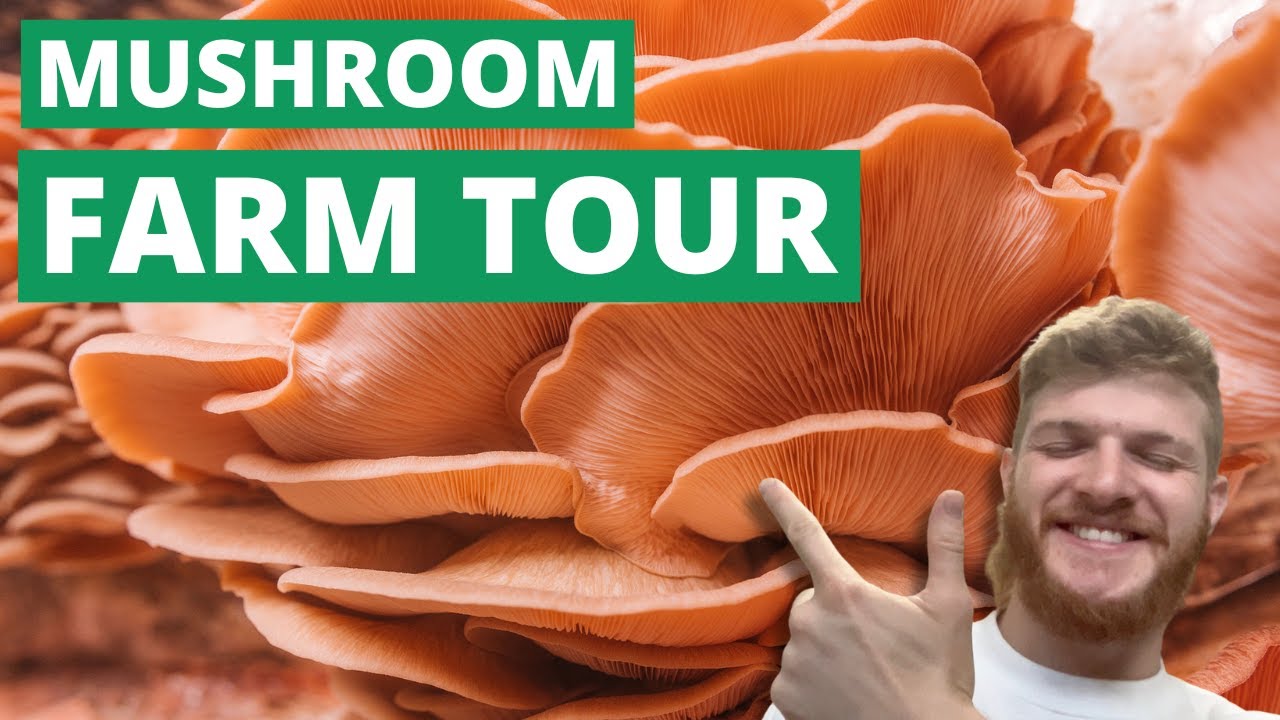The image is a panoramic, digital advertisement featuring a vibrant and intricate close-up of peach-colored coral mushrooms. These mushrooms dominate the background, with their curling layers and striations vividly visible from a side and underside perspective, stretching across the entire viewing area. There are multiple layers, about five or six tall, highlighting the detailed undersides of the primary cluster in the foreground and additional clusters in the background.

In the lower right corner, a slightly out-of-focus inset features a joyful middle-aged man with short blonde hair and a reddish beard. He appears to be smiling with his eyes closed, exuding a teasing yet happy expression. The man is playfully pointing at the mushrooms with his left hand, his fingers forming a V shape, suggesting the large size of the featured mushrooms.

The top left corner of the image has a green banner with blocky white text that reads "MUSHROOM FARM TOUR." The combination of the detailed mushroom background and the cheerful man pointing out the mushrooms enhances the inviting and educational tone of the advertisement.